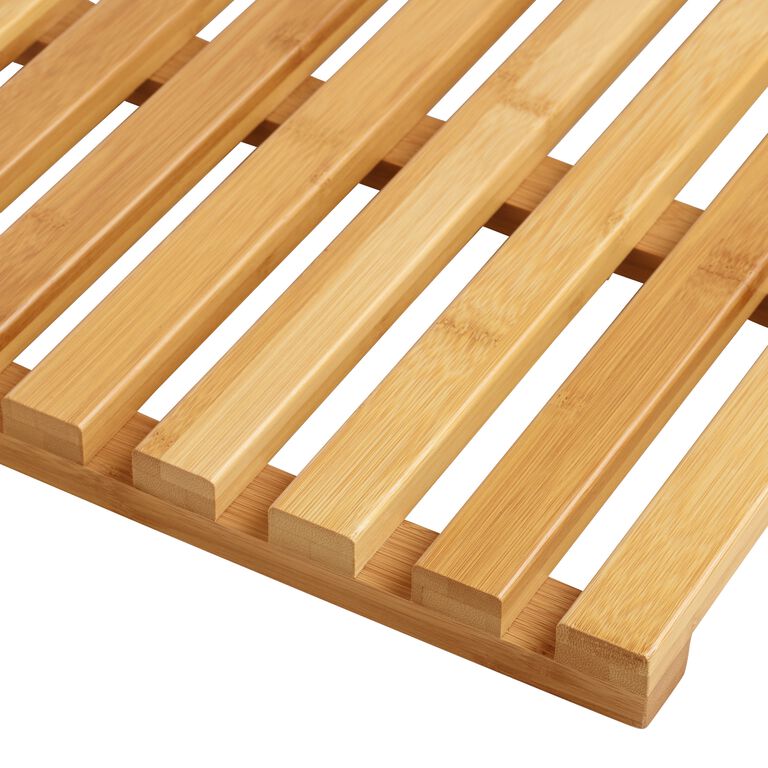This is a detailed close-up photo of a light-colored wooden frame or grate that appears to be a purchasable item, possibly from a catalog. The frame consists of seven or eight vertical wood slats atop two or three horizontal wood beams, forming a grid-like structure. The wood is finely sanded and varnished, showcasing its natural grain and creating a smooth, polished finish in a light tan or bamboo color, with variations between lighter and darker brown tones. The assembly resembles a CHEP pallet or a versatile grate, which could serve multiple purposes such as a drying rack for dishes, a bench base, a shelf, or even a bath mat to stand on and let water drip below. The image does not reveal the entire object, making its exact purpose somewhat ambiguous.